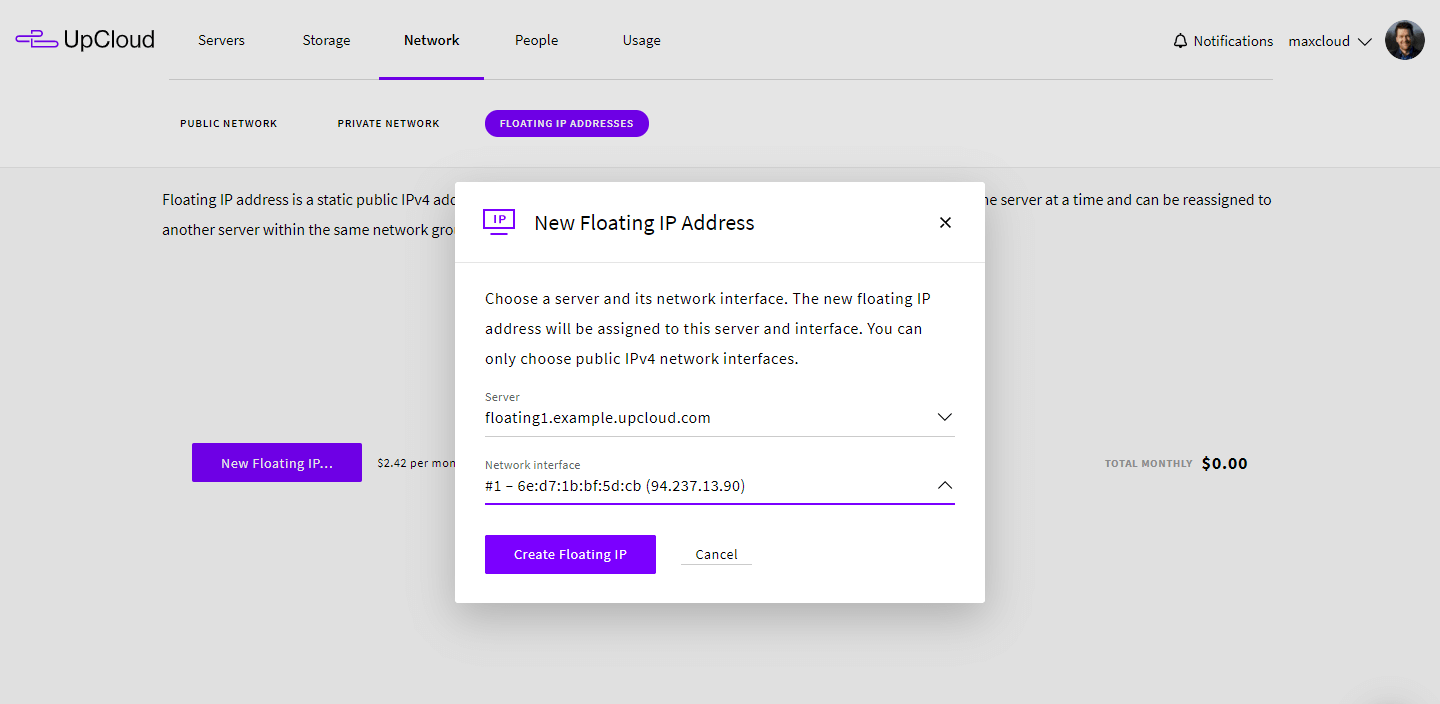This image is a screenshot captured from a PC or laptop, showcasing the user interface of the UpCloud website. In the upper left-hand corner, the UpCloud logo is prominently displayed, featuring a distinct purple squiggly line beside the name "UpCloud" written in black text with capitalized initials 'U' and 'C'. The background of the interface is clean and predominantly white.

The website navigation bar is visible, providing clickable tabs labeled: Server, Storage, Network, People, and Usage, allowing users to navigate through different sections of the platform.

Centrally positioned on the screen is a prominent white pop-up prompt box that contrasts with the slightly dimmer background. The pop-up is titled "New Floating IP Address." Below the title, the instructions read: "Choose a Server and its Network Interface. The new floating IP address will be assigned to this server and interface. You can choose any public IPv4 network interfaces."

The pop-up contains two sections, each equipped with drop-down menus for user input. At the bottom of the pop-up is a noticeable purple button labeled "Create the Floating IP," inviting users to finalize the process.